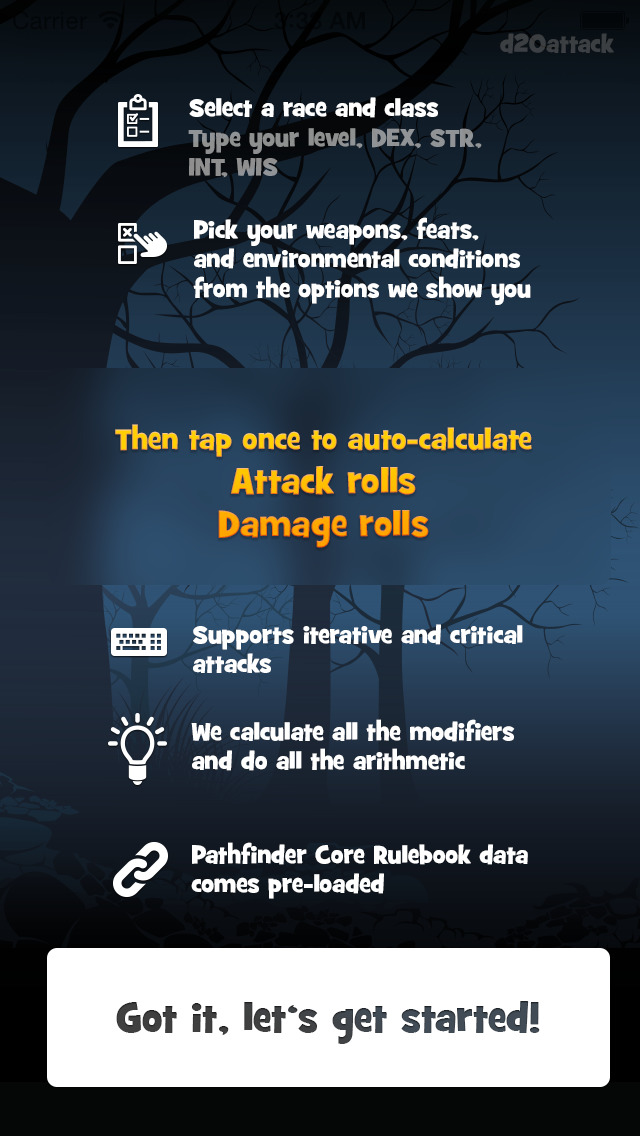Here's the cleaned-up and detailed caption for the screenshot image:

---

The image appears to be a screenshot from a mobile game set against a night sky backdrop sprinkled with mist and featuring eerie, leafless trees reminiscent of a Halloween theme. In the upper right corner, three such trees add to the haunting ambience. In translucent gray font in the upper corner, it reads: "d20 Attack."

Centrally positioned in white font, the text states: "Select Race and Class." To the left of this text, there is a clipboard icon.

Below this, an instructional prompt in gray font says: "Type Your Level, DEX, STR, INT, WIS." Just beneath that, the white text advises players to: "Pick Your Weapons, Feats, and Environmental Conditions from the Options We Show You." Adjacent to this message, on the left, is an icon featuring a human hand pressing a button.

Further down, a translucent rectangle blends with the night sky background. Within this rectangle, a yellow font instructs: "Then tap once to auto-calculate attack rolls, damage rolls." Underneath this, the white text reads: "Support iterative and critical attacks," accompanied by a keyboard icon. The message continues explaining: "We calculate all modifiers and do the arithmetic," adjacent to a light bulb icon.

Finally, at the bottom of the screenshot, a line of text in gray font informs the user: "Pathfinder Core Rulebook data comes preloaded," next to a chain icon.

---

This detailed caption should provide a comprehensive description of the screenshot's contents.